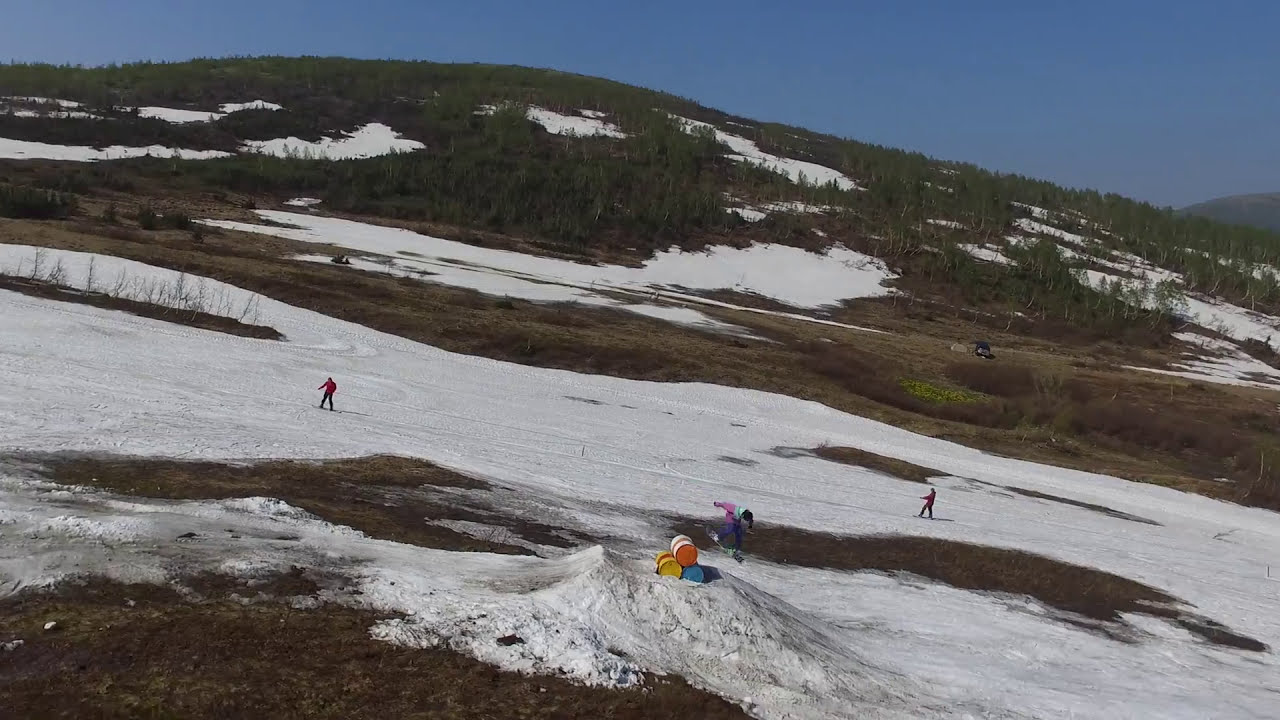In the image, a lively scene of people engaged in snowboarding and skiing unfolds on a mountain that appears to be in the transitional phase of early spring. The mountain terrain is a mix of patches of white snow and exposed brown dirt, indicative of the changing seasons. In the foreground, a prominent snow jump is in the center, adorned with colorful barrels in orange, yellow, blue, and white. A snowboarder is captured midair above the jump, executing a thrilling maneuver. Flanking this central figure, additional snowboarders can be seen in the background—one to the right and another to the left—each seamlessly gliding down different sections of the slope.

Surrounding the action, green trees and sparse patches of snow dot the mountain side, with some areas already beginning to reveal grass and the earthy tones beneath. The scene is vibrant and dynamic, further amplified by the varied attire of the snowboarders and skiers, who sport coats in colors like red and pink, contrasted by their black pants. Above, the sky stretches in a clear, uninterrupted blue, framing the entire picturesque outdoor setting. The barrels and intermittent snowy patches add splashes of color and texture to the slope, culminating in a captivating snapshot of winter recreational activities against a backdrop of natural beauty.